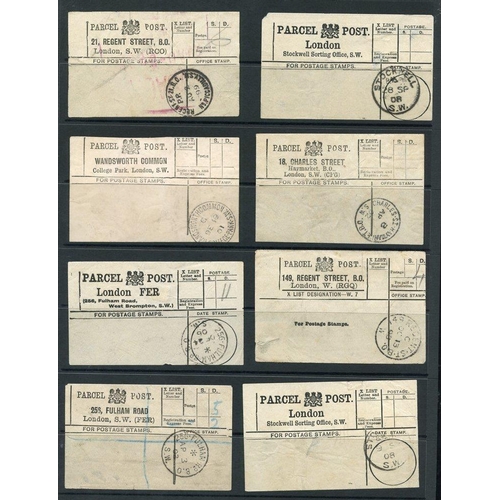This detailed image features a collection of eight vintage parcel post receipts, meticulously arranged in two neat columns of four. Each receipt, reflecting an old-fashioned, handwritten style, is nestled within a clear pocket against a black background, accentuating their aged and historical appearance. Every receipt prominently displays "Parcel Post" and specifies various London addresses, differing in details but unified by their stamps placed in the lower right corner. Starting from the top left, the addresses include:

1. Parcel Post, 21st Regent Street, London.
2. Parcel Post, Wandsworth Common, College Park, London.
3. Parcel Post, London F.E.R.
4. Parcel Post, 25 Fulham Road, London Southwest.

In the second column, from top to bottom:

5. Parcel Post, London Stockwell Sorting Office.
6. Parcel Post, 18 Charles Street, Haymarket.
7. Parcel Post, 149 Regent Street.
8. Parcel Post, London Stockwell Sorting Office.

These receipts, each showing signs of their time with handwritten notes and postal marks, offer a glimpse into the historic parcel post system of London.